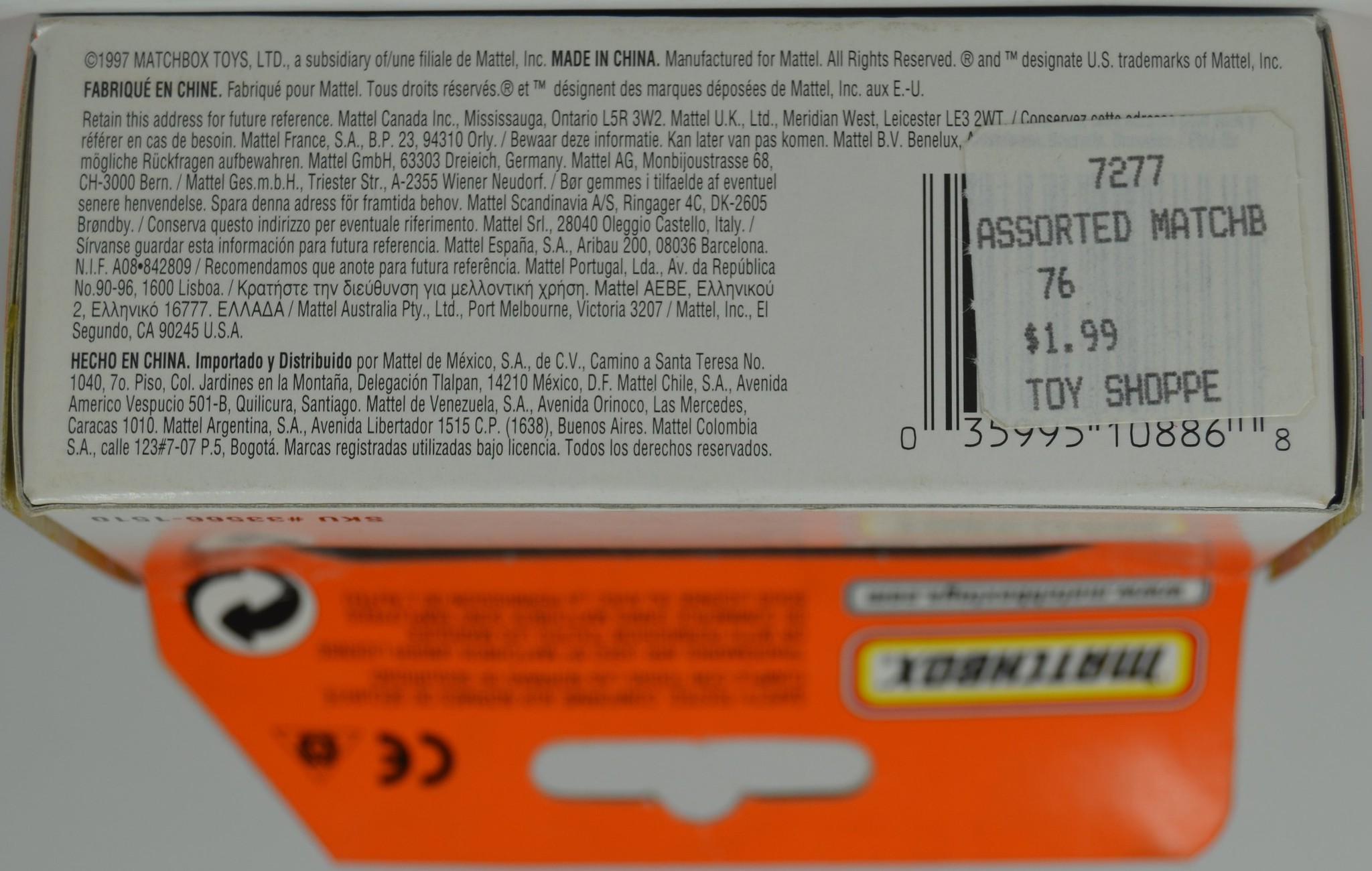This image showcases the bottom of a packaging for a Matchbox toy car. The packaging consists of a white cardboard box displaying various pieces of information. Attached to the cardboard is the signature orange-colored Matchbox box, designed for retail display with a tab for hanging. The tab prominently features the Matchbox logo along with the distinctive orange branding. 

A sticker placed over the UPC reads: "7277 Assorted Match B76 $1.99 at Toy Shop." The packaging also includes detailed manufacturing information: "1997 Matchbox Toys LTD, a subsidiary of Mattel, made in China, manufactured for Mattel, all rights reserved, and designated US trademarks for Mattel Inc." Additional information is presented in various other languages, likely reiterating the previously mentioned details.